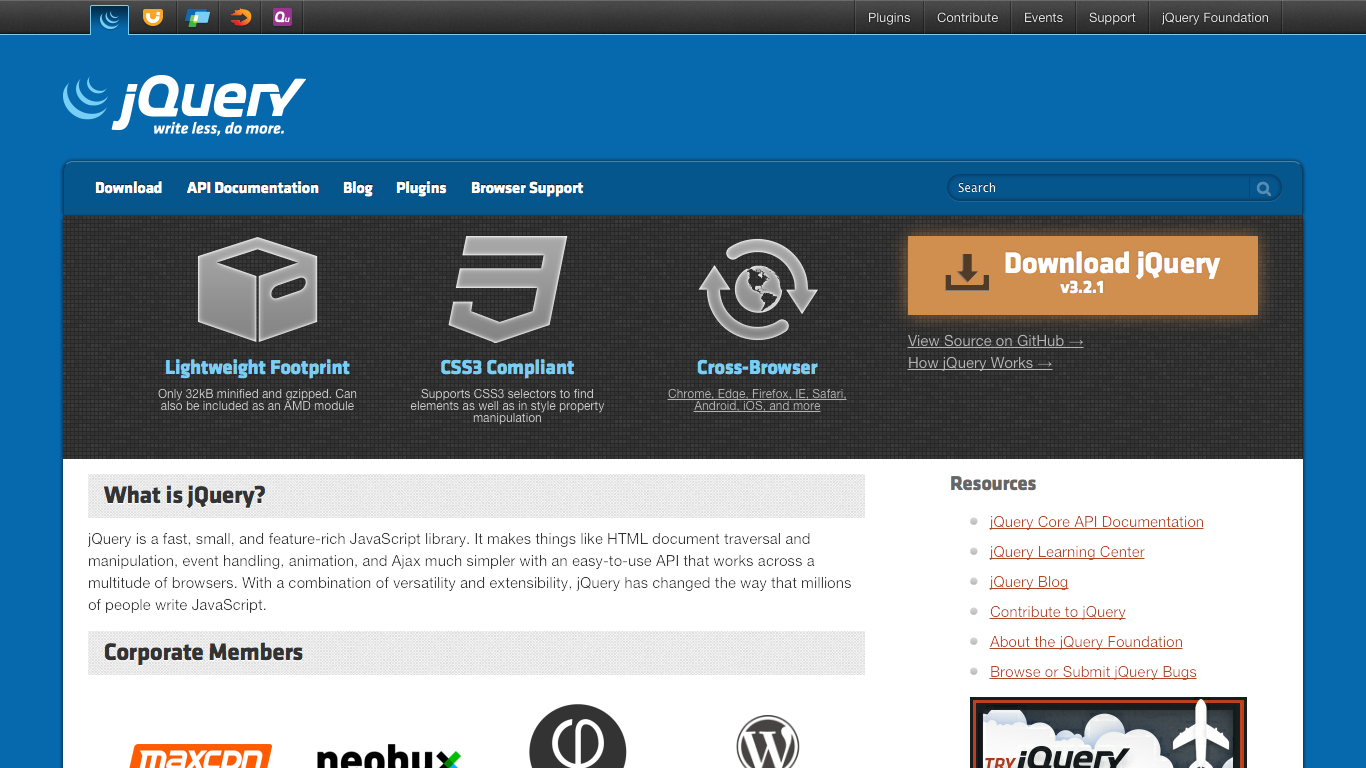The image is a screenshot of a website. At the top left corner, the word "jQuery" is prominently displayed alongside the tagline "Write Less Do More." Below this header, there are several navigation tabs or categories. The first tab is labeled "Download," followed by "API Documentation," "Blog," "Plugins," and "Browser Support." On the far right side of the header, there is a search bar with the placeholder text "Search."

Below the main header, there are three distinctive icons, each associated with a feature of jQuery. The first icon, labeled "Lightweight Footprint," depicts a file drawer, symbolizing the minimal code needed for jQuery. The second icon, labeled "CSS 3 Compliant," features a shield-like design, indicating that jQuery adheres to CSS 3 standards. The third icon, labeled "Cross-Browser," shows a globe with two arrows encircling it, representing jQuery's compatibility with multiple web browsers.